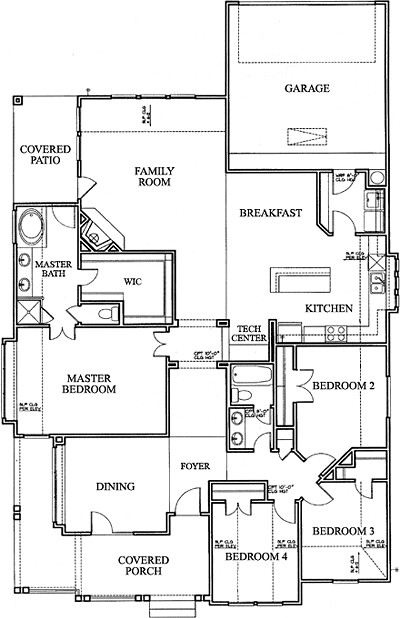This is a detailed top-down diagram of a rectangular house plan, showcasing a meticulously labeled layout of various rooms in black text, suggesting an early architectural design stage.

In the top-right corner, a large square represents the garage. Below the garage to the left is the breakfast and kitchen area, with designated countertops and a stovetop. Moving further down is Bedroom 2, followed by Bedroom 3 in the bottom-right corner and Bedroom 4 directly to its left. Centrally located on the bottom edge, connected by small stairs, is a labeled covered porch.

Continuing left from the covered porch, the foyer is situated adjacent to the dining room on the lower left corner. Above the dining room is the master bedroom, the largest sleeping area besides the garage. North of the master bedroom, the master bath takes place on the left side with detailed placements of sinks, bathtubs, showers, and toilets. To the right of the master bath is a section labeled "WIC" (Walk-In Closet).

In the top-left corner of the house, a covered patio is situated. Moving right from the patio, the largest internal room labeled family room completes the layout, emphasizing the house's practical and detailed design for future architectural development.